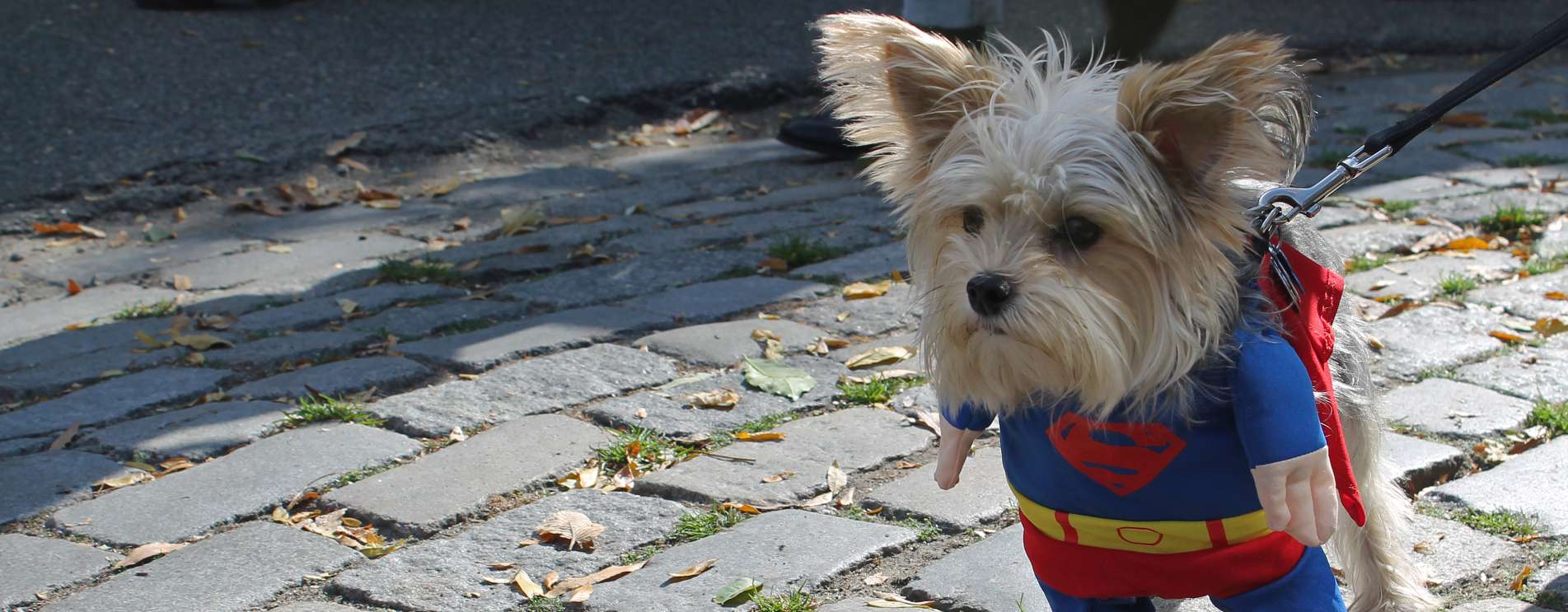In this photograph, we see a small, white, furry dog positioned slightly right of center, with its head turned to the left, showcasing a serious expression. The dog, which appears to be a tiny toy or pocket breed, has two small ears that are brown on the interior and white on the exterior, sticking out to the right and left. Its distinctive black button nose and black eyes peek out from its furry face. The dog is wearing a Superman outfit, with its head where Superman's head would be, making it look like the dog is embodying the superhero. To the right of the dog, there is a metal attachment connected to a black leash, stretching up and off the image in the upper right-hand corner, indicating the dog might be tethered. In the background, there's a gray brick surface with grass and dry leaves growing between the bricks, suggesting an outdoor setting. Additionally, towards the top middle of the image, a human foot is partially visible.